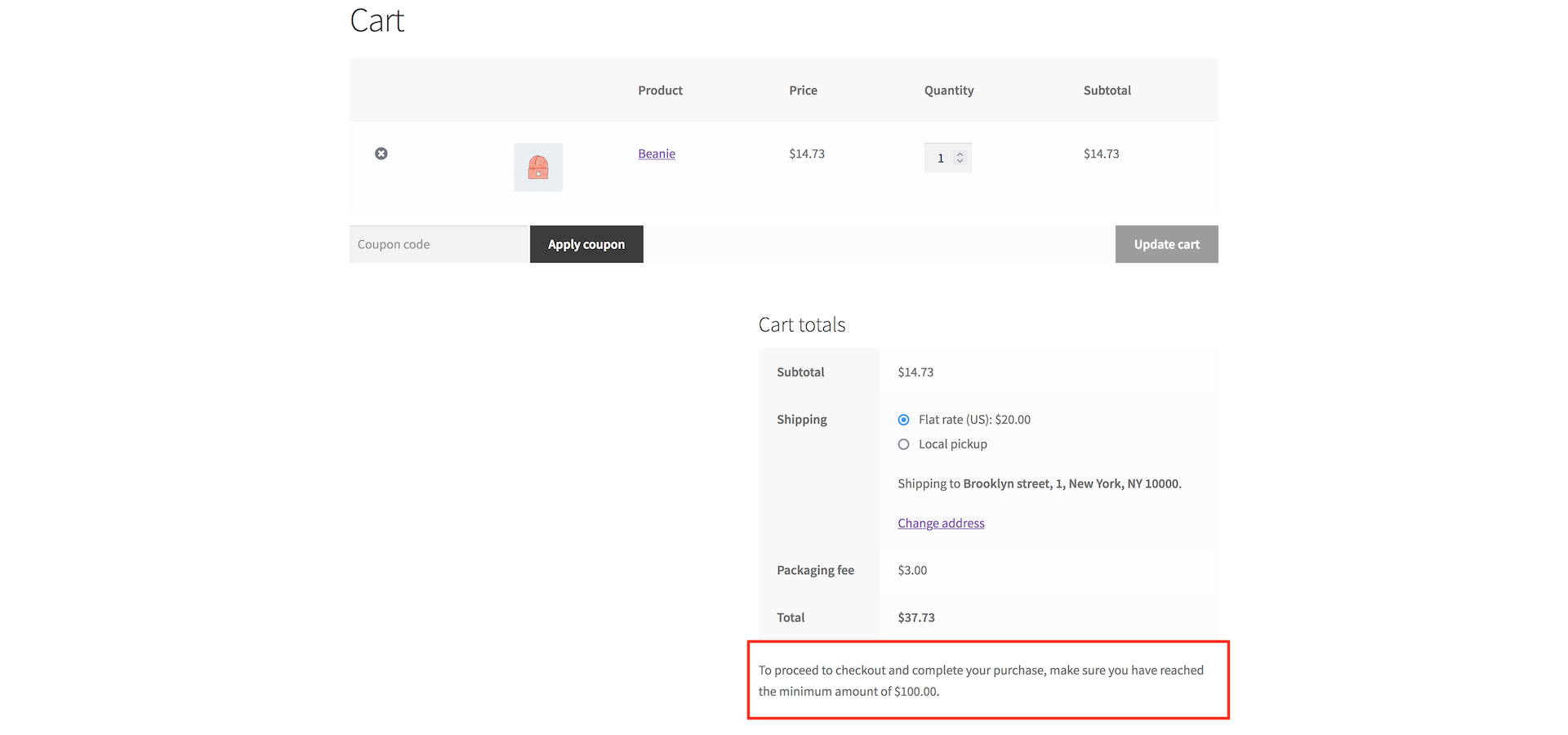This is a detailed screenshot of a website showing a shopping cart pop-up menu. The background is white, and at the top of the pop-up, the word "CART" is prominently displayed in black font. Below this header, there is a gray rectangle containing the headers: "Product," "Price," "Quantity," and "Subtotal."

Beneath the headers, in a white rectangle, there's a small, unclear photo of an item. Next to this photo, under the Product column, the word "Beanie" appears in blue, indicating a clickable link. Adjacent to this, under the Price column, is "$14.73." Under the Quantity column, the number "1" is displayed, and under the Subtotal column, the amount "$14.73" is shown.

Further down, another gray rectangle contains fields and buttons labeled "Coupon Code," "Apply Coupon," and "Update CART." Beneath these, there's a gray square labeled "CART Totals," detailing a breakdown of costs: "Subtotal: $14.73," "Shipping: Flat Rate U.S.: $20, or Local Pickup." The Flat Rate option for $20 has been selected.

The shipping address is listed as "Shipping to: Brooklyn Street, 1 New York, New York, 10086," with a "Change Address" link highlighted in blue. Finally, the summary at the bottom details a "Package Fee: $1," and the "Total: $37.73."